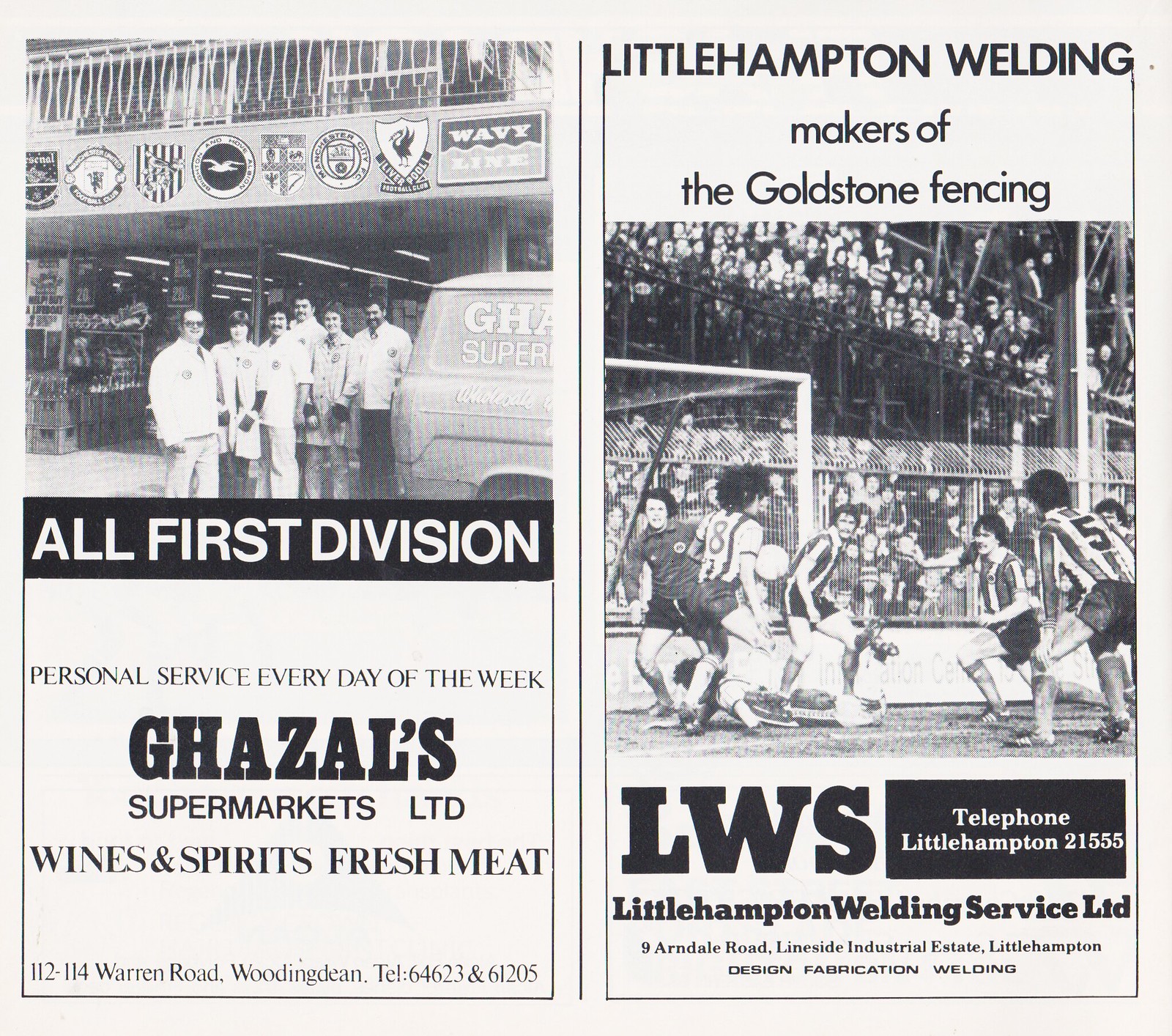In this intricate black-and-white image, the left side displays a group of individuals standing outside a storefront, all dressed in white. Adjacent to them, a partially cropped van is visible. Above the store, signs feature various soccer team logos, including Manchester United, Swansea, and Newcastle, with the store name "Wavy Line" displayed prominently. Below this, a black background with white text reads "All First Division," followed by a white background with black text stating, "Personal Service Every Day of the Week," and more text in larger font proclaiming "Gazelles Supermarkets Ltd," offering "Wines and Spirits Fresh Meat" and located at "112-114 Warren Road, Wooding Dean." The contact numbers "64-623" and "612-05" are also provided.

To the right, the image shifts to another advertisement for "Little Hampton Welding, makers of the Goldstone fencing." This segment includes a black-and-white photograph of a dynamic soccer match with six players and a ball center-right, surrounded by numerous spectators both at ground level and in elevated stands. In large black font, the acronym "LWS" is highlighted next to contact information, "Telephone Little Hampton 21555." Further text describes "Little Hampton Welding Services, LTD" at "9 Arndale Road, Lineside Industrial Estate, Little Hampton," specializing in "Design, Fabrication, Welding."